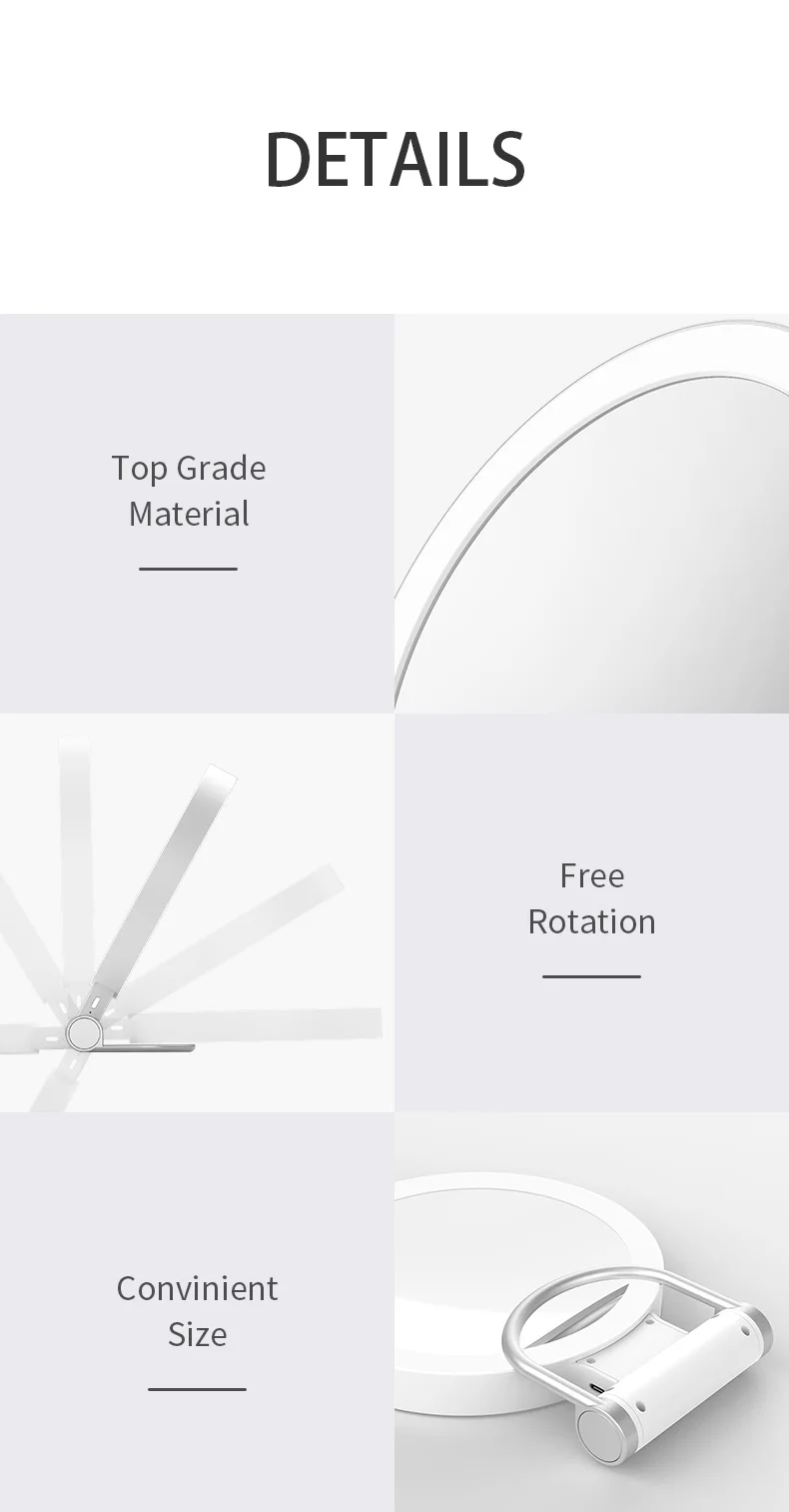At the very top center of the image, the word "DETAILS" is prominently displayed in bold, black text. Below this, the image is divided into multiple sections.

In the top left square, the background is light gray. Inside this square, the words "Top Grade Material" are written in black text and are underlined with a small black line beneath them. Adjacent to this text, there is a long, white curved object shaped somewhat like a rainbow.

Descending below this section, to the left, there is a white circle with long gray lines radiating outward.

To the immediate right of the first square, the next section also has a light gray background. Here, the words "Free Rotation" are displayed in black text, also underlined for emphasis.

In the bottom left corner, another light gray box contains the phrase "Convenient Size" in black text, which is also underlined.

To the lower right of this section, there is a depiction of a white object with a silver hook at one end, possibly resembling a lock or similar device. This object appears to be approximately four inches long and is displayed within a light gray box.

Overall, the image uses a combination of light gray backgrounds and black text to detail the features and characteristics of the subjects within each section.